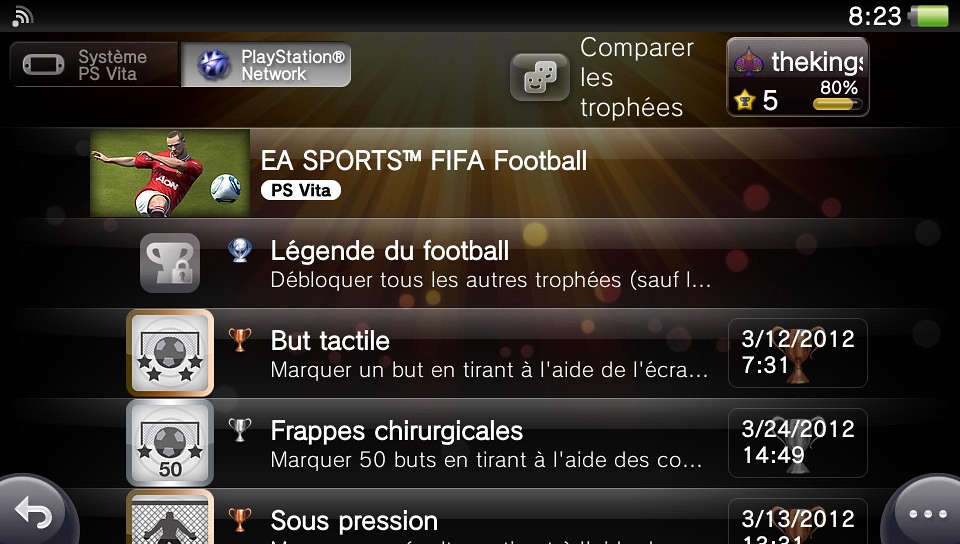The image depicts a screenshot from a handheld PlayStation device, likely a PS Vita, showcasing a user interface predominantly in French. On the top left, the tab for the PlayStation Network is selected, while to its left, the "System" and "PS Vita" indications are visible. The screen includes a connectivity logo on the upper left and the time, 8:23, along with a battery icon on the upper right, adjacent to the option "Comparer les Trophées" (Compare Trophies). The central segment of the screen features a list of horizontally stacked menu options with black, white, and gray bars, each representing different game titles. The highlighted row shows "EA Sports, FIFA Football, PS Vita," complete with an icon of a soccer player kicking a ball. Beneath it are options for "soccer legend," "Boot Actile," and "Frappes Chiruricales." At the bottom left, there's a back arrow to return to the previous screen, and at the bottom right, three dots to access more options. The overall background is black, emphasizing the sleek design of the interface.